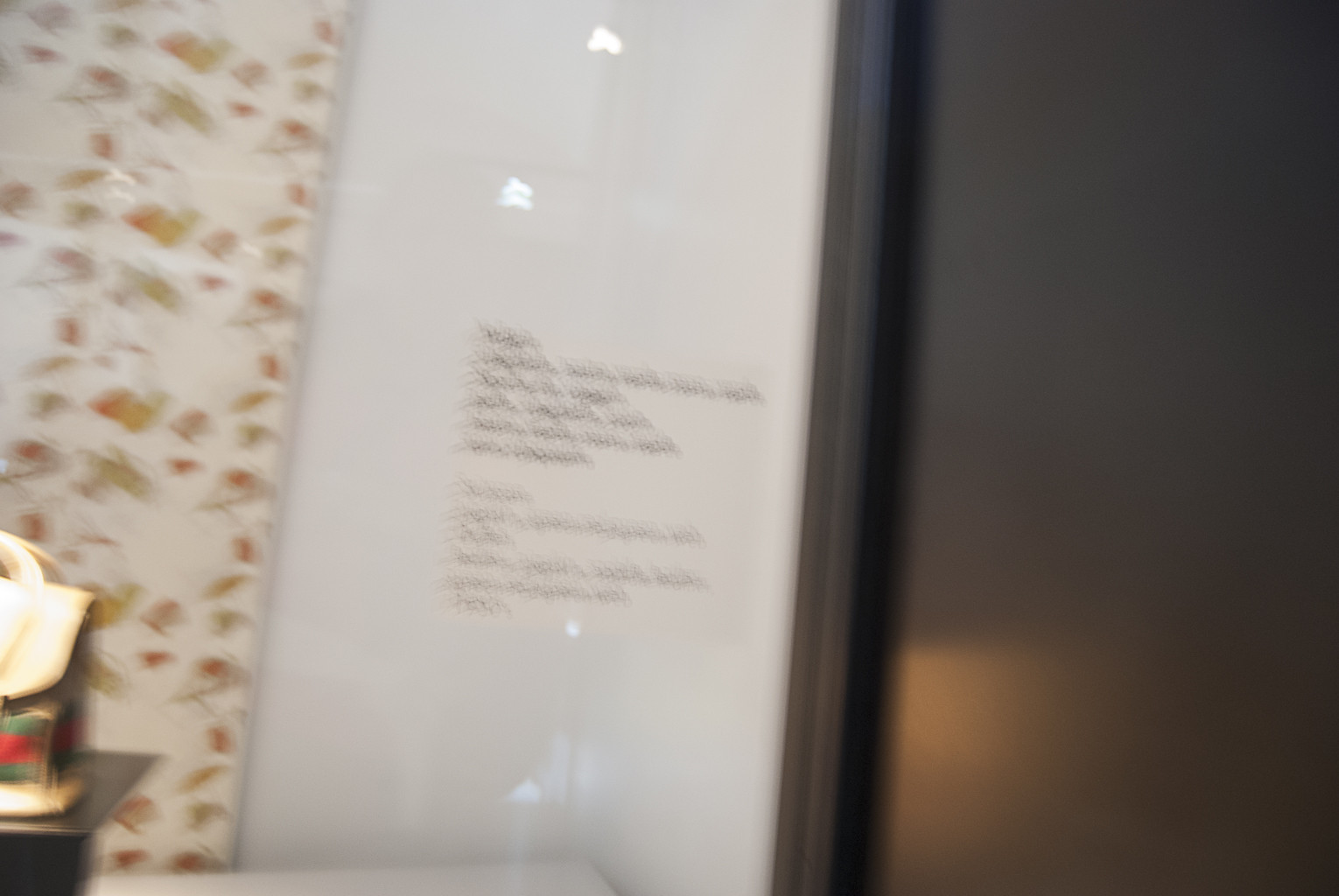The image captures a severely out-of-focus scene dominated by a white wall at its center. To the left, a floral-patterned wallpaper extends from the top to the bottom, partially obscured by a dark wooden side table on which an indiscernible bag rests. To the right is what appears to be a black door, though only half of it is visible and the handle is not discernible. The focal point on the white wall is a square poster board with black, handwritten text, though the blurriness renders the message unreadable. The poster could potentially be mounted on a refrigerator, adding to the ambiguity of the scene.